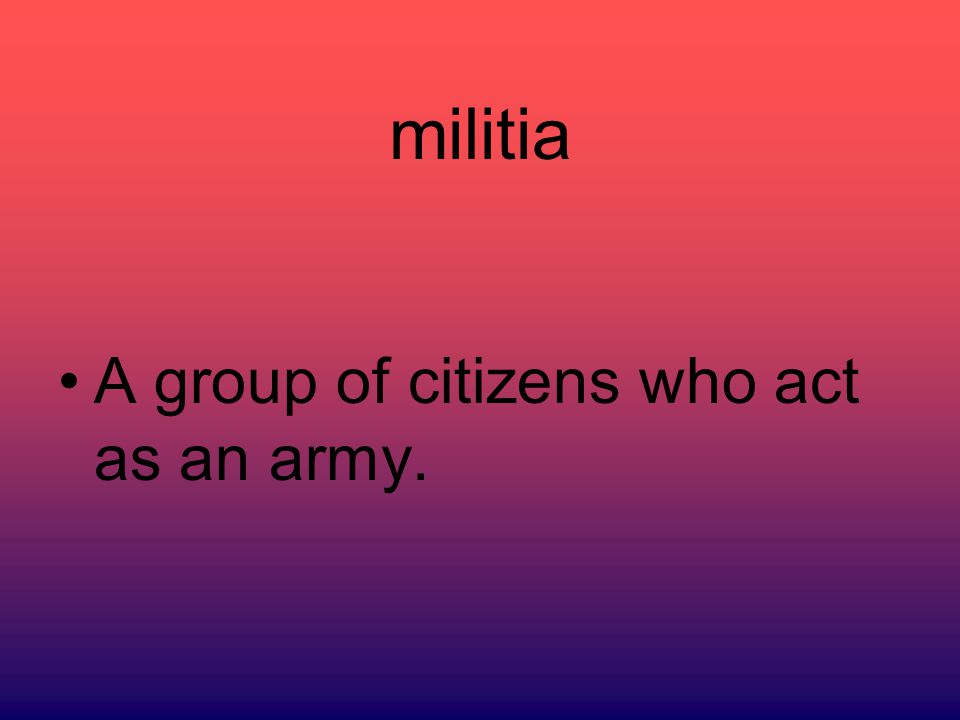The image depicts a slide from a PowerPoint presentation with a visually appealing background that transitions from a gradient red at the top to blue-purple at the bottom, with shades of purple in between. At the top of the slide, in lowercase black text, the word "militia" is written in a simple, modern, and thin font. Beneath this heading, also in black text but in proper case starting with a capital 'A', is the definition: "a group of citizens who act as an army." The word "militia" is positioned in the red portion of the gradient, while the definition is primarily set against the purple shade. This setup creates a striking visual effect that blends the colors harmoniously from top to bottom.